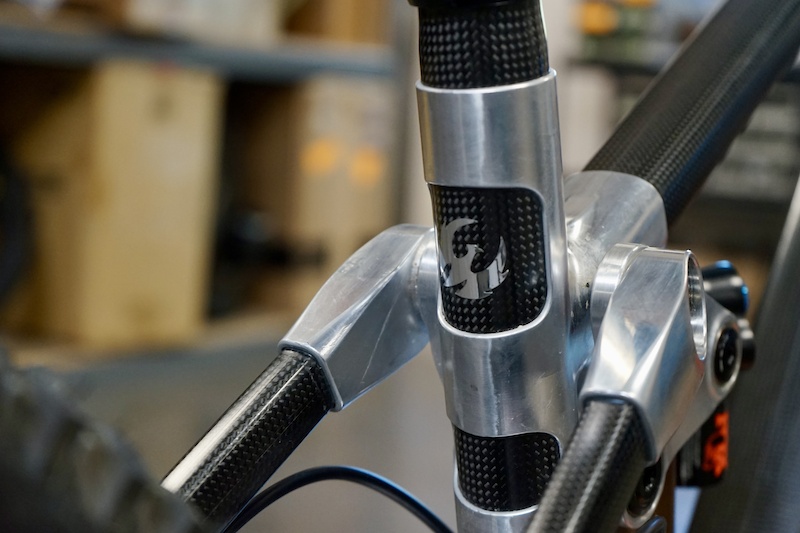This close-up photograph captures the front fork and head tube of a high-end bicycle. Dominated by gunmetal gray and black carbon fiber components, the frame showcases a prominent silver Phoenix logo at the center. Aluminum or stainless steel fittings, along with visible cables and calipers, hint at the bike’s advanced construction. The background is blurry, suggesting an indoor setting that could be a warehouse or a bicycle store, where indistinct shapes of shelves, boxes, and possibly a staircase are faintly discernible. The photograph focuses solely on this intricate section of the bicycle frame, leaving out details like pedals, handlebars, or the complete structure.